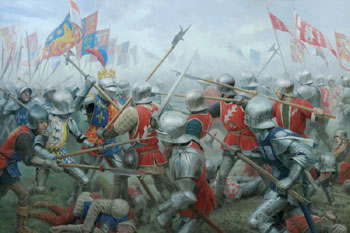This small square image is a detailed painting depicting a chaotic battle scene. The battlefield is crowded with numerous soldiers, all clad in suits of armor and wearing silver helmets. The majority of the soldiers, especially those on the right, are adorned in red tunics, while some on the left appear to be in blue. The ground beneath them is a dusty expanse of dirt, adding to the gritty atmosphere. 

In the upper sections of the image, various flags are prominently displayed: on the left, the flags boast a mix of red, blue, and yellow colors, while on the right, the flags are distinctly red. 

Among the soldiers, several are armed with spears, pushing aggressively towards the left side. Scattered across the dirt, a few soldiers lie motionless, adding to the grimness of the battle. The sky overhead is laden with smoke and clouds, casting a gray, misty pall over the scene, which recedes into the background where more soldiers continue to clash.